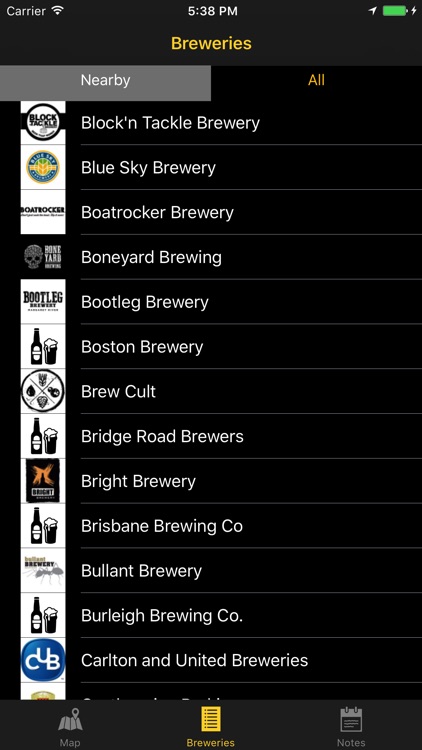This image is a screenshot of an iPhone app displaying a list of breweries. The top banner shows 'carrier' with a full connection icon on the left, the time as 5:38 PM in the middle, and a full, green charging battery icon with an electricity symbol on the right. Below this, the yellow text "Breweries" is centered. Underneath, there are two tabs: 'Nearby' on the left (selected and gray) and 'All' on the right (unselected and black). The screen has a black background, with a list of breweries displayed in white text. Each brewery name is accompanied by an app icon on the left. The breweries listed alphabetically from top to bottom include Block and Tackle Brewery, Blue Sky Brewery, Boat Rocker Brewery, Boneyard Brewing, Bootleg Brewery, Boston Brewery, Brew Cult, Bridge Road Brewers, Bright Brewery, Brisbane Brewing Co., Bullitt Brewery, Burleigh Brewing Co., and Carlton and United Breweries. At the bottom of the screen are three icons: a map icon on the left, a breweries icon (highlighted in yellow) in the middle, and a notes icon on the right.